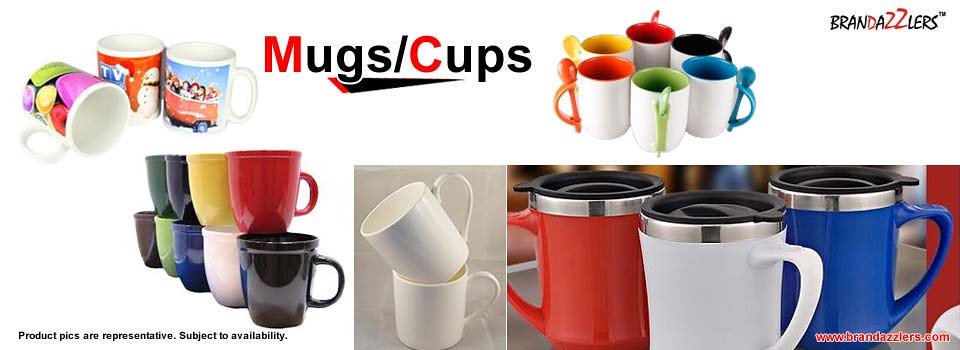This advertisement for Brandazzlers mugs and cups is a vibrant and colorful display that features a variety of travel mugs in blue, red, and white, as well as standard mugs with either solid colors or playful designs such as balloons and snowmen. Primarily, the travel mugs are equipped with black spill-proof tops, ideal for on-the-go use. The image is horizontally oriented and prominently features the header "Mugs/Cups" at the top, alongside the brand name and availability information. Below the header, some mugs and cups are notably scattered, adding a casual, lively element. Additionally, the display includes white mugs with coordinating colored handles and spoons, emphasizing the brand's commitment to personalization and fun shapes. The text in the ad clearly states that the products are "representative and subject to availability," and a website address is provided for further details.